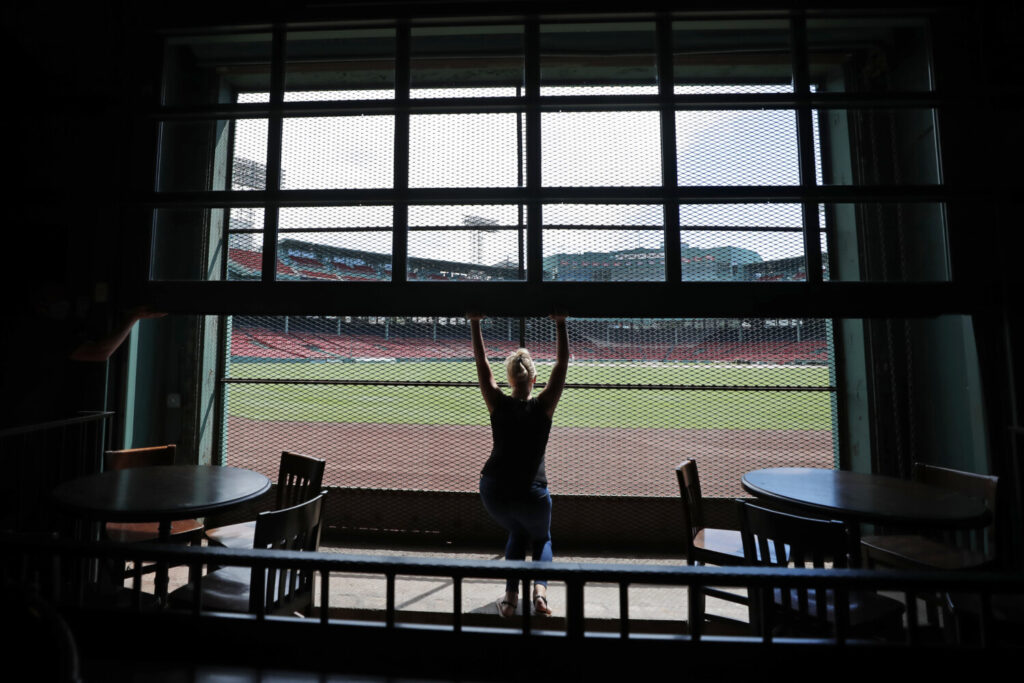A photograph captures a woman with blonde hair from behind as she stands inside a dimly-lit stadium cafe, surrounded by round wooden tables and matching wooden chairs with slatted backs. The woman, dressed in jeans and a tank top, is lifting a large, see-through glass garage door, allowing light to flood in from the green baseball field outside. The empty stadium, which can accommodate thousands of spectators, contrasts with the serene indoor setting where the light brown flooring adds warmth. The woman appears silhouetted as she opens the door, possibly to let in air, with the fenced seating outside indicating the close proximity to the baseball field. The overall ambiance suggests the end of a day, with the stadium quiet and the cafe preparing to close.